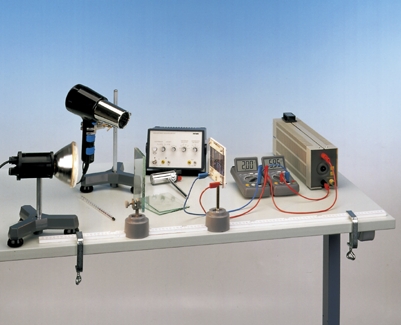The photograph depicts a detailed setup on a rectangular wooden table with black metal legs. The scene primarily includes various electronic devices arranged meticulously, indicating an experimental setup. Prominently towards the right, two voltmeters, connected with red and blue wires, display readings, and are interlinked with other electronics, one possibly a printed circuit board mounted on a base with a whiteboard. A spotlight on a tripod is positioned on the far left, directed towards the devices, while near the spotlight, a handheld hair dryer is aimed at the equipment, suggesting a testing process. Clamps hold some components securely. The background features blue and gray hues with a black-framed picture adding to the backdrop. The predominant colors of the objects are black, gray, and white. The overall arrangement of seven objects, mostly electronic devices, is meticulously orchestrated, underscoring a precise and possibly scientific experimentation environment.